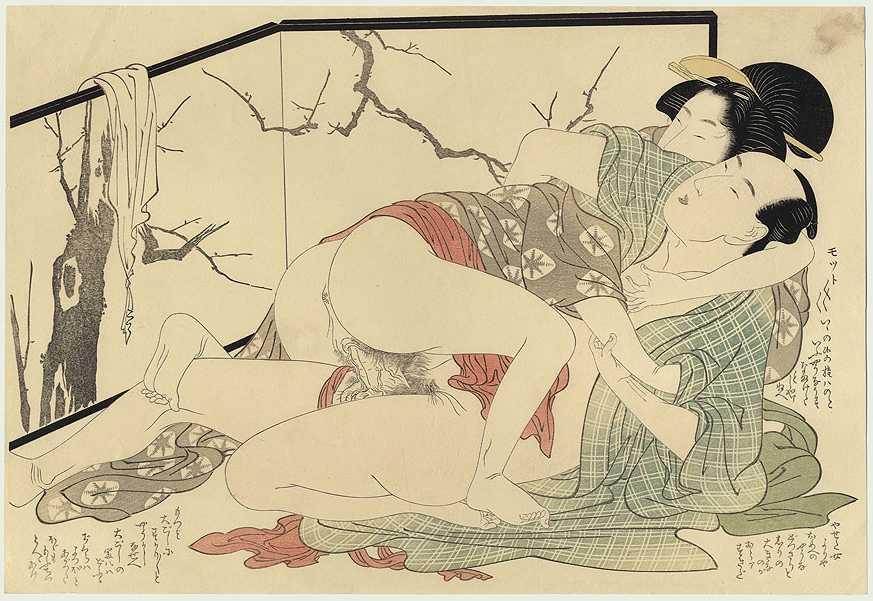The image is an intricate and explicit artistic depiction, reminiscent of traditional Japanese or Chinese styles, portraying an intercoursing couple. The couple, dressed in ornate, decorative gowns with intricate Asian prints, are depicted in a highly unusual sexual position: the woman, sporting an elaborate hairstyle adorned with a large gold comb and chopsticks, is squatting on top of a balding man. Both figures are facing opposite directions, appearing to have each other in a headlock, with the woman's arms wrapped around the man. Seen in muted tones of sepia, grey, white, with splashes of red and blue, the background features a screen adorned with what seems to be tree branches. Scattered clothing lies on the floor behind them and there's Japanese or Chinese text in the bottom corners of the artwork. The setting also includes artistic elements like a bamboo-like wall with a black border.